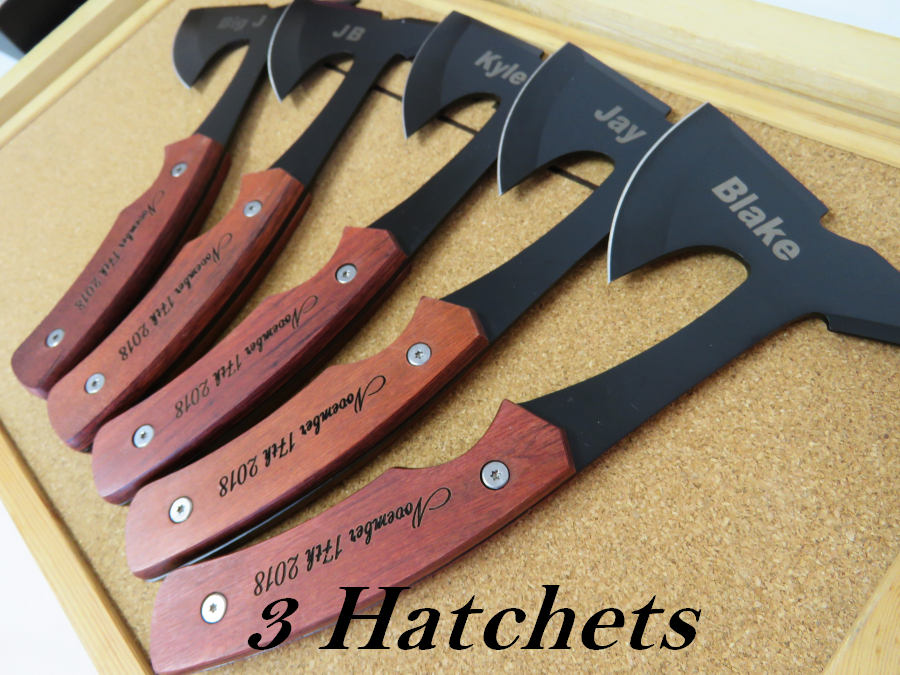This image features five hatchets, each with black blades and brown wooden handles, neatly arranged in a row on a beige corkboard-like surface, elevated at a 45-degree angle. At the bottom of the image, the phrase "three hatchets" is printed in black font, occupying roughly a tenth of the image space. The hatchet heads are marked with names in white: Big J, JB, Kyle, J, and Blake. Each handle is engraved with the date "November 17th, 2018" in cursive near two silver screws. The arrangement suggests a display, possibly for an event such as a hatchet-throwing competition or a commemorative ceremony.